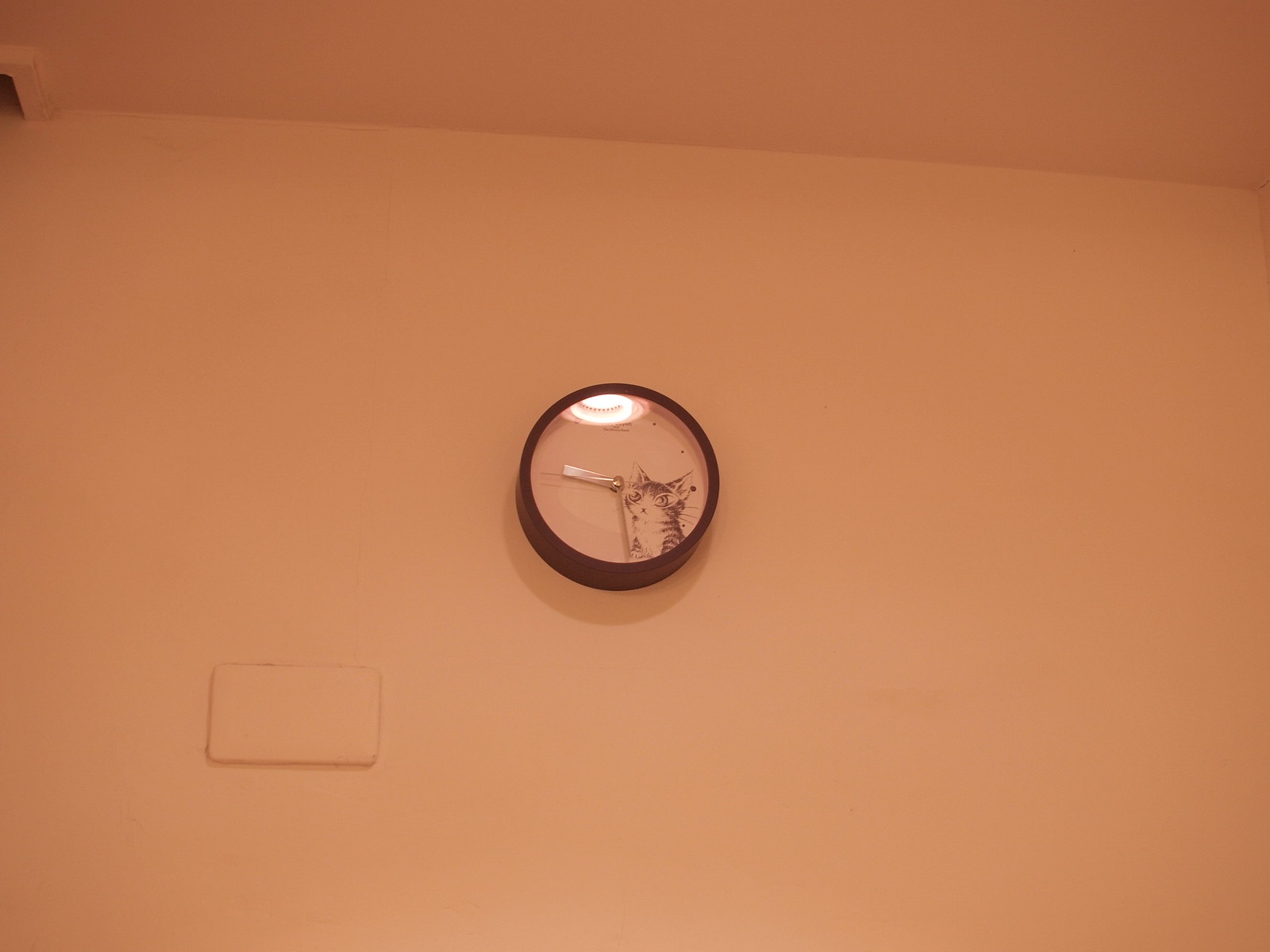This indoor photograph captures a prominent round clock mounted on a plain white wall. The clock features a substantial outer frame finished in a dark brown hue, which adds a touch of sophistication to its design. The clock face is minimalist with a clean white background, detailed with small dots marking each hour. Silver hands gracefully indicate the time. What sets this clock apart is the charming addition at the bottom right corner: a picture of an inquisitive kitten with stripes and a white front, appearing to peek up from the edge of the clock face, its gaze fixed curiously on the clock hands. This whimsical touch adds an element of playful interest to the otherwise simple wall decor.